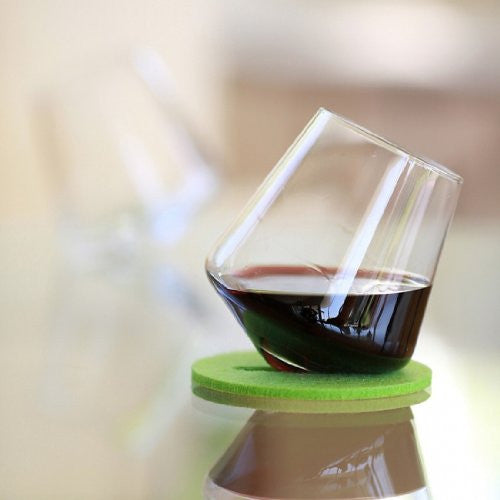This meticulously staged photograph captures an artsy glass of red wine, positioned on a brown trapezoid-shaped stand. Atop the stand are two coasters—a nude-colored one beneath a green one—providing a layered surface for the wine glass. The glass is intentionally designed to lean at a sharp angle which gives the impression that it might tip over. Its cut-glass design and the way it refracts light adds an intricate, eye-catching detail. The wine, filling about one-third of the glass, appears deep red to purple in color. The scene is illuminated by bright lighting, likely from a photographer's studio setup, further enhancing the glass’s reflective quality. The background includes a blurry image of another identical, empty glass leaning in the opposite direction, and both glasses cast reflections as if they are placed on a glass surface. The composition creates a dramatic, almost surreal visual effect that draws the viewer's attention to the unique design of the angled glassware.